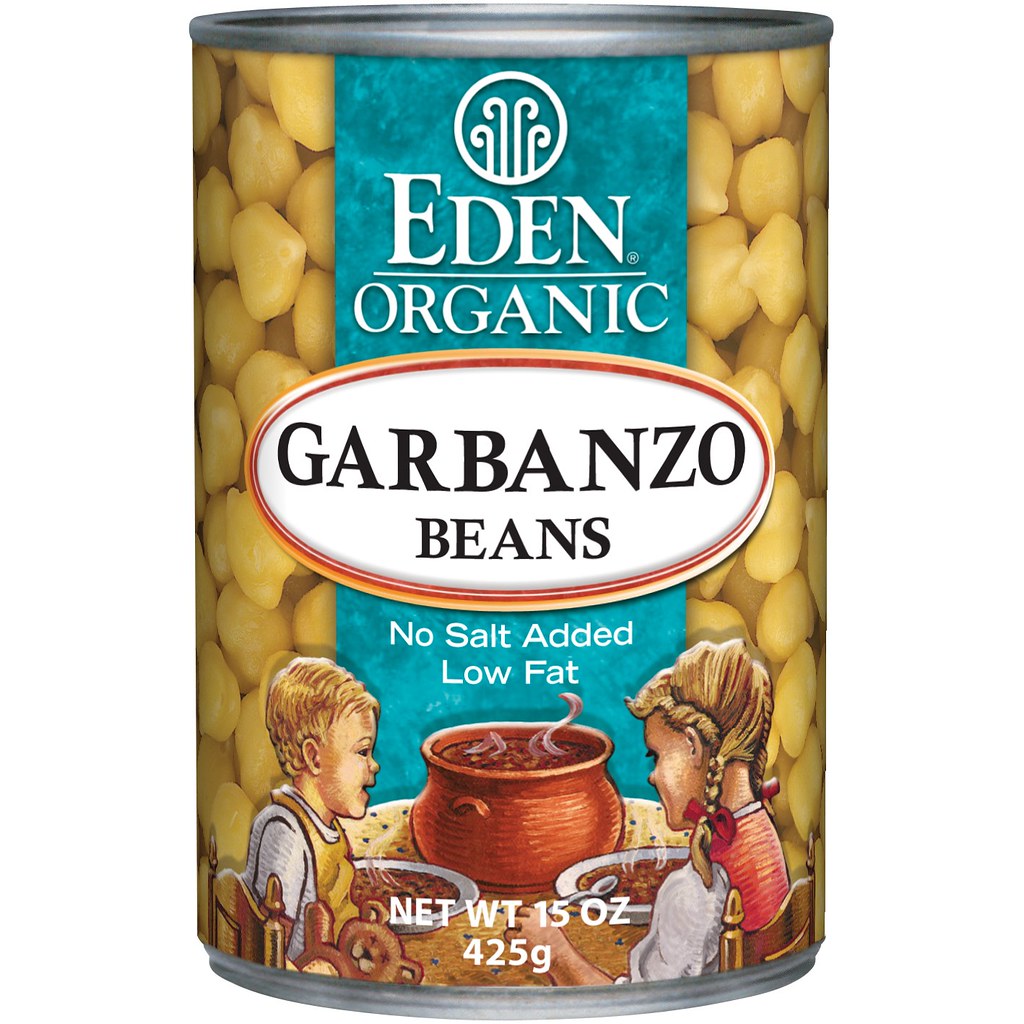This image showcases a can of garbanzo beans from the Eden Organic brand. The label on the can teems with intricate details and vibrant colors. Dominating the label is a central turquoise strip where "Eden Organic" is prominently displayed. Below this, nestled within a large oval outlined in red and gold, the words "Garbanzo Beans" are written in black text on a white background. Notable features also include the statements "No Salt Added" and "Low Fat" printed alongside the oval.

On both sides of this central band, the label features realistic images of garbanzo beans, portraying the product inside. Additionally, there is a charming illustration of two children seated at a table. One child is in the act of spoon-feeding the other, who is eagerly awaiting their turn. In the backdrop, a large pot with steam wafts upward, suggesting that the garbanzo beans are being cooked. The label also mentions the net weight and the number of grams, completing the extensive detailing of this organic product's packaging.